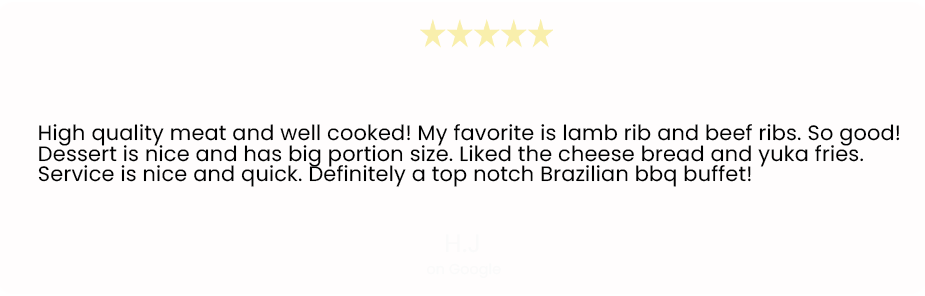The image is minimalistic, featuring a clean layout with a white background. At the top center of the image, there are five small, yellow stars, indicating a five-star rating. Beneath these stars is a considerable amount of blank space, creating a clean and uncluttered appearance. 

Following this blank space, there is a succinct restaurant review written in black, sans serif text. The review reads: "High quality meat and well cooked. My favorite is lamb rib and beef ribs. So good. Dessert is nice and has big portion size. Liked the cheese bread and yucca fries. Service is nice and quick. Definitely a top notch Brazilian BBQ buffet."

The text itself is centered, maintaining the simple and straightforward aesthetic of the image. The review consists of seven sentences and is followed by more blank space at the bottom of the image, emphasizing the clear and focused presentation of the content. There are no other images, text, or elements on the page, ensuring the viewer’s attention is solely on the glowing review and the five-star rating.